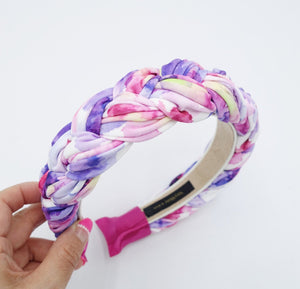The image is a close-up of a multicolored, tie-dye headband that features a braided pattern of light pink, dark pink, purple, blue, red, and white hues. The inner portion of the headband, which appears to be made of tan or white fabric, is visible on the right side and contains a pink felt section, presumably for better grip on the head. The headband is being held in the lower left corner by a hand with pink nail polish, showcasing the knuckle and a partly plain, partly pink fingernail. The background of the image is a gradient of white to lightish blue.